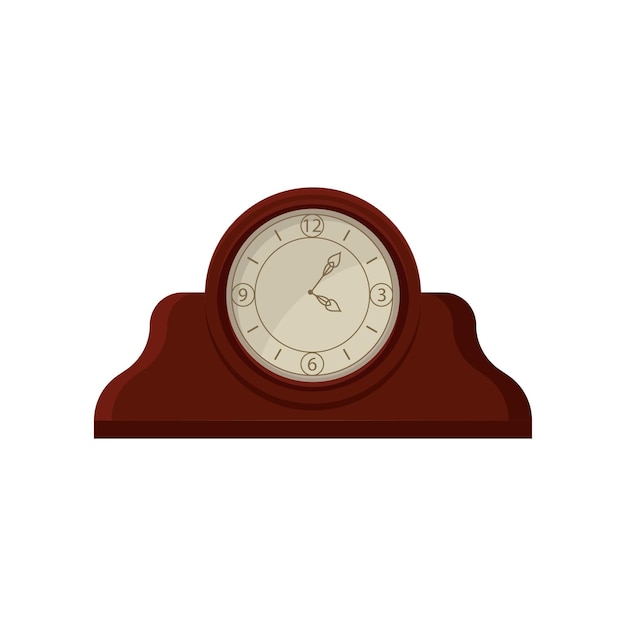This digital illustration depicts an old-fashioned mantel clock set against a white background. The clock features a deep cherry red frame and a slightly curved rectangular wooden base, rendered in three shades of brown for a blocky effect. The clock face is white with brown hands, and it prominently displays the numbers 12, 3, 6, and 9, each encased in a thin circle. Between these numerals are simple mark ticks indicating the other hours. The time is shown as 4:05, with the hands styled as lines ending in arrow shapes. The clock's design is reminiscent of traditional analog clocks, blending simplicity with a touch of nostalgic artistry.